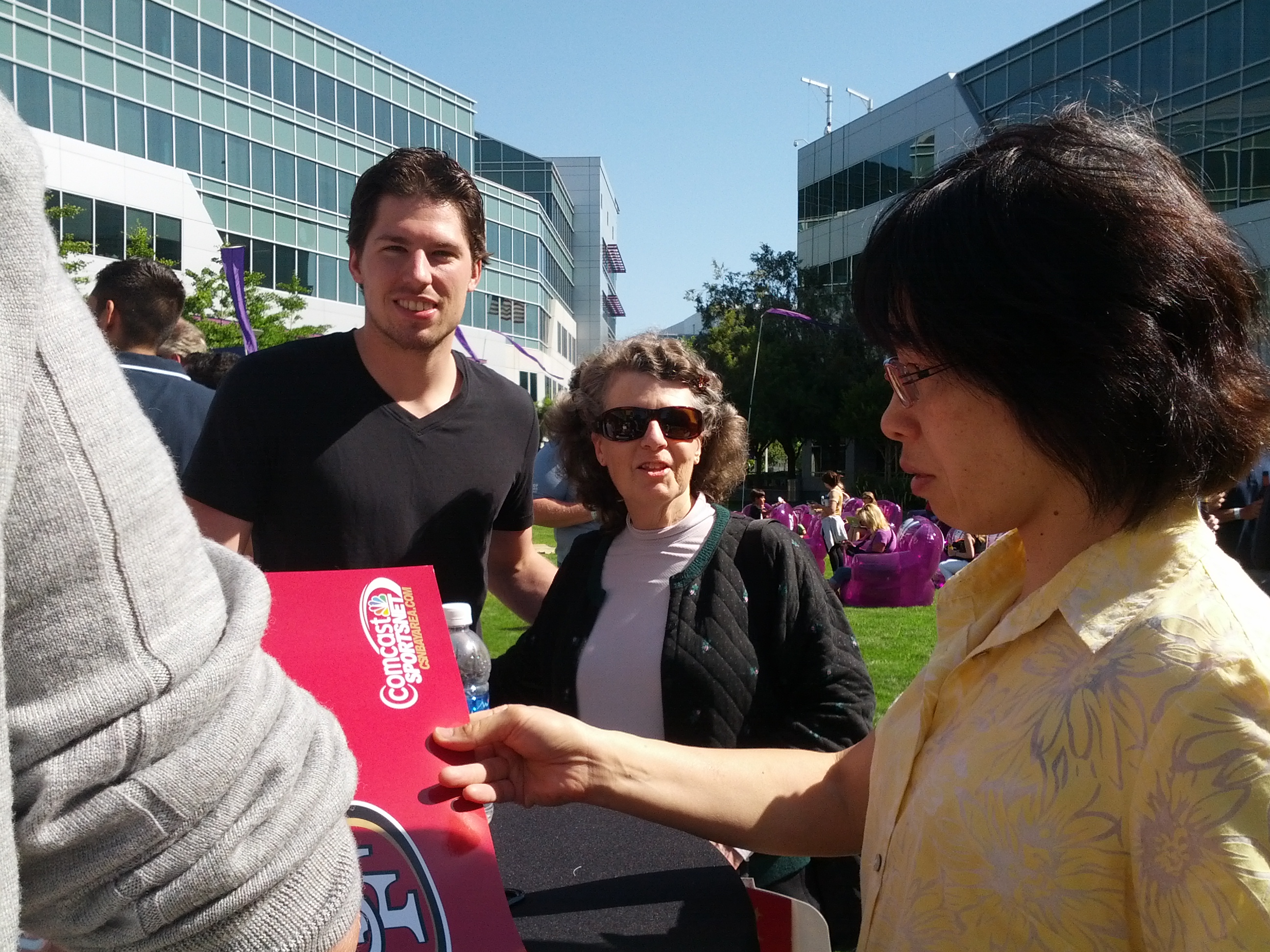In this bright and sunny outdoor image, two very tall buildings with all-glass windows form the backdrop. In the foreground, three individuals are prominently visible, with the upper halves of their bodies clearly shown. Among them, a woman on the right stands out, wearing a yellow blouse adorned with gray and white flowers. She has shoulder-length black hair and wears glasses. Holding a red sign that reads "Comcast SportsNet," with a symbol for the San Francisco football team, she faces to the left. 

Next to her, an older woman, possibly in her 50s or 60s, has shoulder-length curly brown hair with some gray streaks and dons a white shirt under a black jacket. To her left, a smiling young man with short dark hair is seen wearing a black, short-sleeve V-neck t-shirt. 

In the left-hand side of the picture, the arm of another person, clad in a gray sweater, is also visible. Behind this group, several people are leisurely seated on purple inflatable chairs on a green lawn. The combined details from these multiple descriptions come together to provide a vivid and comprehensive depiction of the scene.